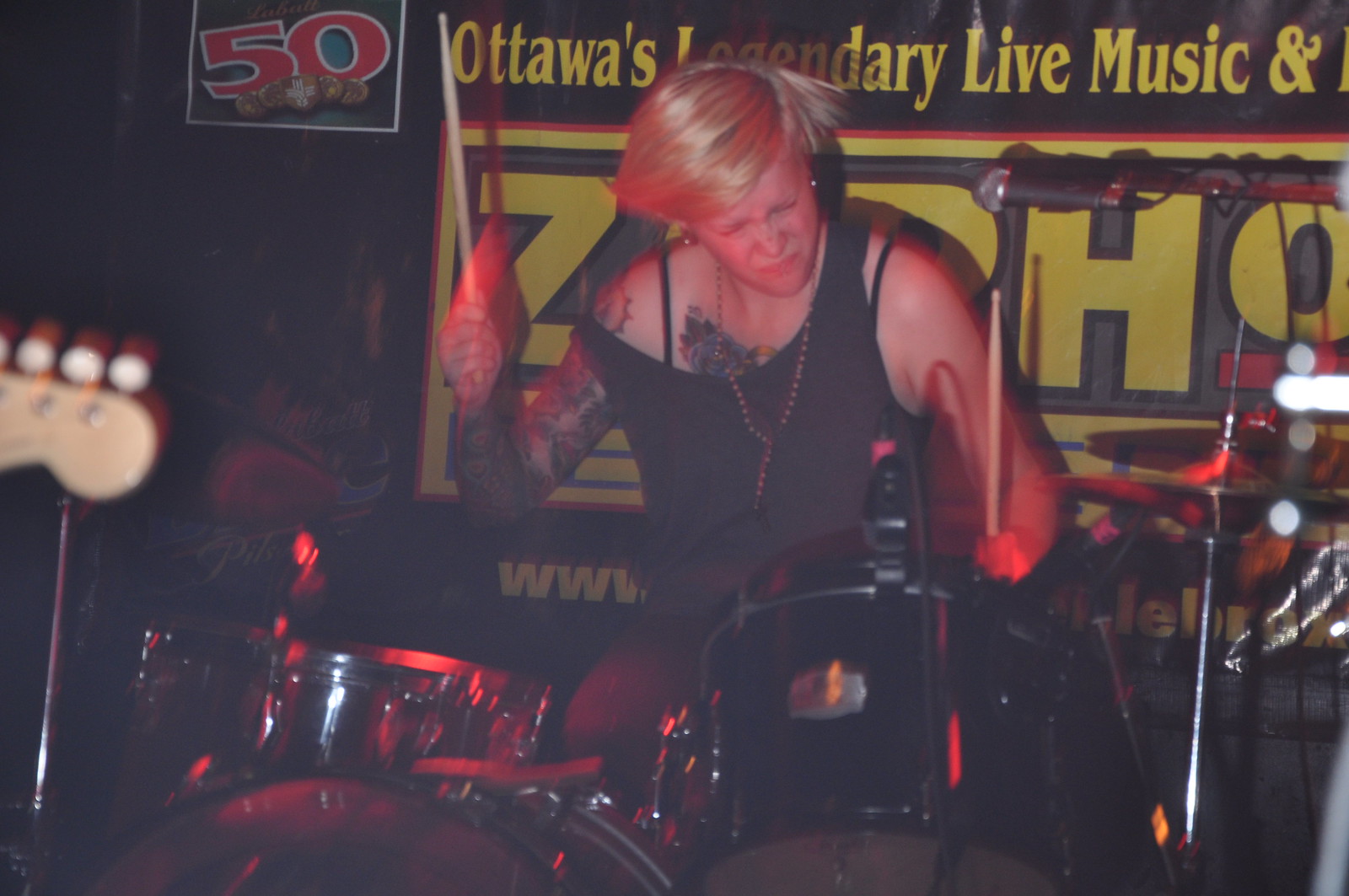The photograph captures the intense, energetic moment of a female drummer deeply engrossed in her performance. Framed in a horizontal rectangle, the image positions her slightly off-center to the right, set against a very dark, possibly black background that highlights her presence. Dressed in a slightly skewed black tank top exposing black bra straps and adorned with tattoos on her left arm and chest, she exudes a rock-and-roll aura. Her bright blonde hair, in motion, suggests the vigor with which she plays, her head swaying rhythmically. Her eyes are squeezed shut, emphasizing her deep connection to the music. She grips drumsticks in both hands, poised mid-action over a dark drum set at the bottom of the frame. A microphone stand flanks her right side, while the tip of a guitar, played by an off-screen band member, is visible on her left. Behind her, a banner with yellow and red details reads, "Ottawa's legendary live music and..." partially obscured by her fervent drumming. The image, illuminated with touches of yellow, red, silver, beige, black, and white, is taken indoors on a band stage, capturing the raw essence of a live music performance.